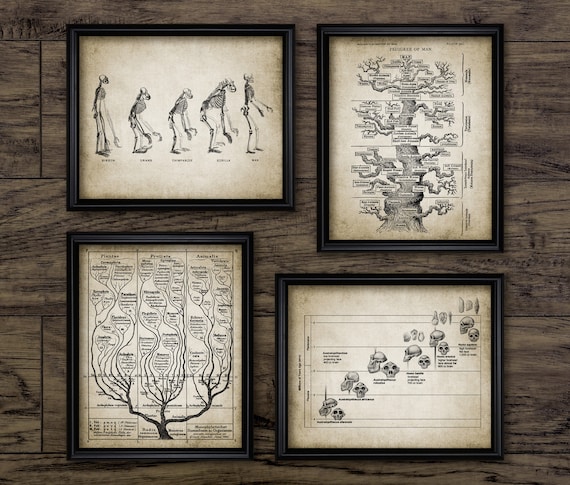This photograph captures four framed, vintage-style pen and ink illustrations, each displayed in elegant black frames against an off-white background. The top left image features a series of human and related hominid skeletons, possibly illustrating aspects of human evolution though not in chronological order. The top right frame contains a detailed tree diagram with numerous small, unreadable labels. The bottom left illustration showcases the morphological changes in primate skulls over time, while the bottom right image is another tree diagram with extensive, yet unclear text labels. These meticulously arranged frames rest on a polished wooden floor, exuding a sense of classical scholarly presentation.